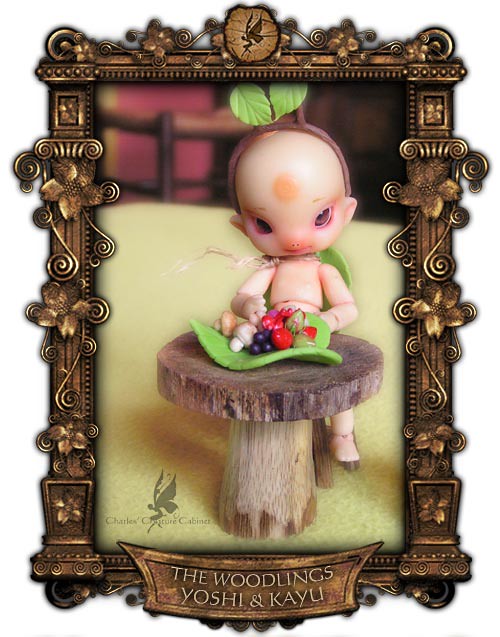The image is a computer-generated graphic featuring an elaborately detailed and irregular bronze or brass frame adorned with fish heads, flowers, pillars, vines, and squiggles. At the top center of the frame is a circular emblem showcasing a butterfly logo, which is repeated in profile at the bottom left corner of the image. Below the emblem, a banner with raised text reads "The Woodlings, Yoshi, and Caillou." 

Within the frame, set against a cream-colored background, sits a figure resembling a Kewpie doll. The character has a large head with almond-shaped eyes angled sharply away from the nose, giving an alien-like appearance. The figure's head is adorned with a headband featuring a pair of green leaves. The character, shirtless and with a pinkish-white flesh tone, is seated at a round wood table that looks like a toadstool. On the table lies a large green leaf, upon which assorted mushrooms, strawberries, and blueberries are arranged. A plaque at the bottom of the frame, rendered in the same ornate bronze or brown, reads "Chao's Chocolate Cabinet."